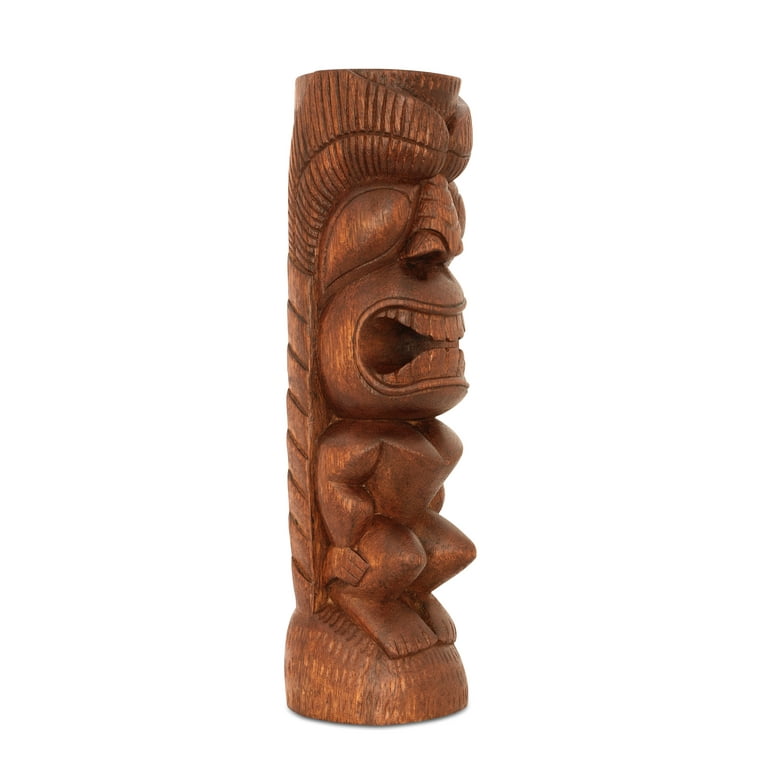In the image, we see a striking sculpture or totem pole carved from a medium brown wood, displaying striations that give it a natural, intricate texture. The sculpture is of a humanoid creature with a disproportionately large head compared to its smaller body. The creature's head, which occupies half the total dimensions, features prominent facial details. It has large, pupil-less teardrop-shaped eyes pointing downwards, a big nose positioned between the eyes, and an open mouth in a fierce grin revealing closely set teeth. Above the eyes, a headdress-like structure adorned with curved lines can be noticed. The humanoid figure is depicted in a squatting posture, with bent knees and arms resting beside its protruding chest. The feet are flat and square, and the entire sculpture, including its round platform base, is carved from a single piece of wood, retaining its natural color.